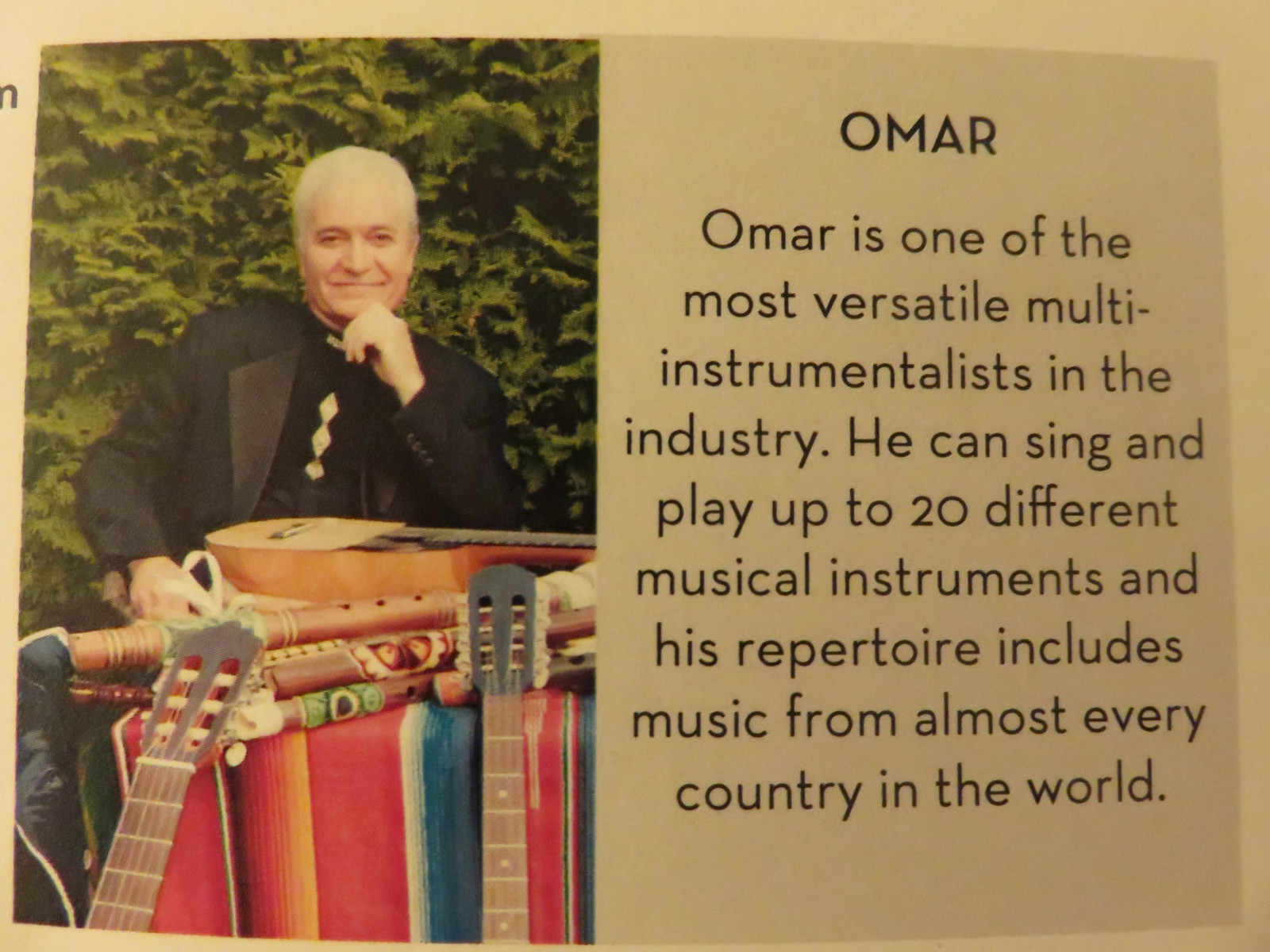This promotional color print features a well-composed photograph of an older gentleman named Omar, renowned for his extraordinary musical talents. Omar, dressed in a black top and a black jacket, appears deeply contemplative with one hand resting thoughtfully on his chin. The background is filled with an array of multiple guitars, highlighting his profound connection to music. On the right side of the print, there is text introducing Omar, emphasizing his status as one of the most versatile multi-instrumentalists in history. The text details that Omar possesses the rare ability to sing and play up to 20 different musical instruments, with a repertoire that spans musical traditions from almost every country in the world. This promotional piece effectively captures Omar's extensive musical expertise and cultural dexterity, inviting viewers to appreciate his remarkable contributions to the world of music.